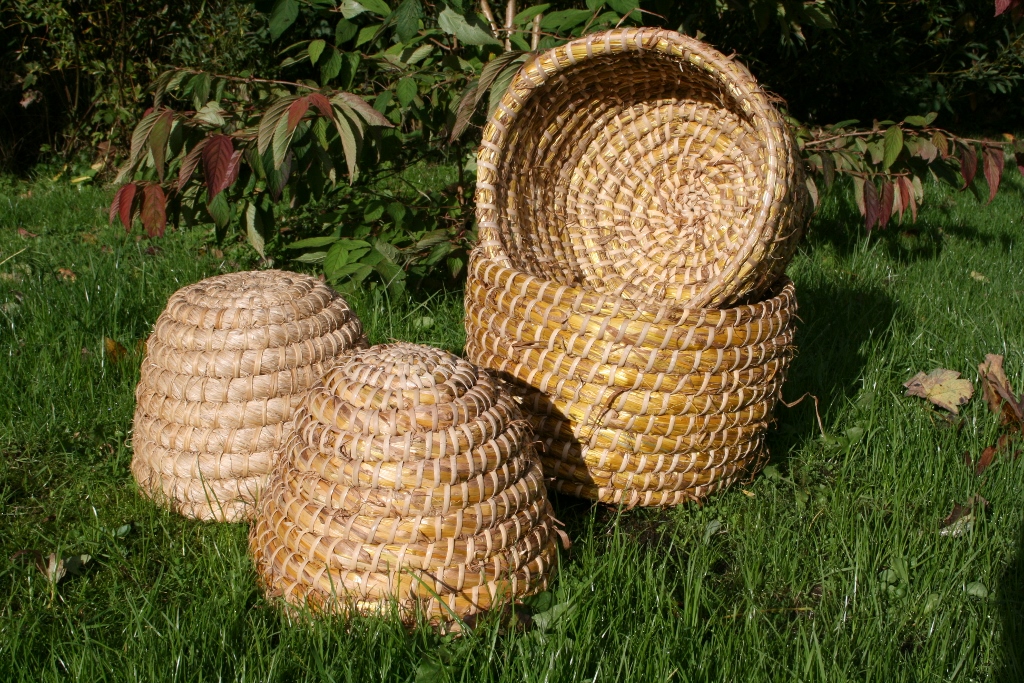This photograph captures a collection of four distinct, handcrafted wicker baskets displayed on lush, bright green grass in a serene yard. The two medium-sized baskets on the left are positioned upside down, with one appearing typical in shape while the other is more cone-shaped, suggesting an artisanal touch. On the right, two larger baskets are staged; the bottom one is placed upright, and a smaller basket leans sideways inside of it, facing the photographer to reveal its intricate interior craftsmanship. The baskets vary in size and shape, reflecting their handmade origins, with noticeable details of brown wicker and beige string work. The background features dense foliage, including trees and bushes, adding to the natural and tranquil setting of the display.